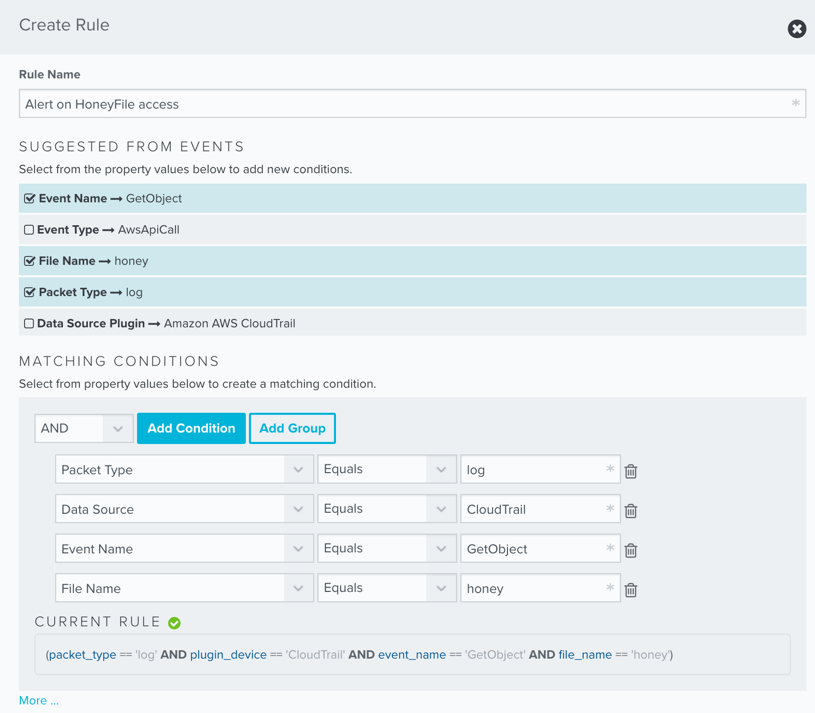The screenshot captures a back-end interface of a website designed to create a new rule. At the top of the interface, there's a heading titled "Create Rule" alongside an exit button located at the upper right corner. Below this heading, a section labeled "Rule Name" is evident, with an entry box filled in with "Alert on Honey File Access."

Following this is a section called "Suggested from Events," which instructs the user to select from the property values below to add new conditions. This section includes several properties such as "Event Name," "Get Object," "Event Type," "AWS API Call," "File Name," "Honey," and "Packet Type," "Log." Notably, "Event Name," "File Name," and "Packet Type" are checked and highlighted in blue.

The next part of the interface is titled "Data Source Plugin" and specifies "Amazon AWS CloudTrail." Further down is the "Matching Conditions" section, directing the user to select from property values below to create a matching condition. This section displays a drop-down menu with the default option "And," accompanied by a blue button labeled "Add Condition" and a white button labeled "Add Group." 

Within the drop-down menus, the configurations are set as follows: "Packet Type" equals "Log," "Data Source" equals "CloudTrail," "Event Name" equals "Get Object," and "File Name" equals "Honey."

At the bottom, the "Current Rule" is displayed, summarizing the conditions: "Packet Type == Log," "Plugin Device == CloudTrail," "Event Name == Get Object," and "File Name == Honey."